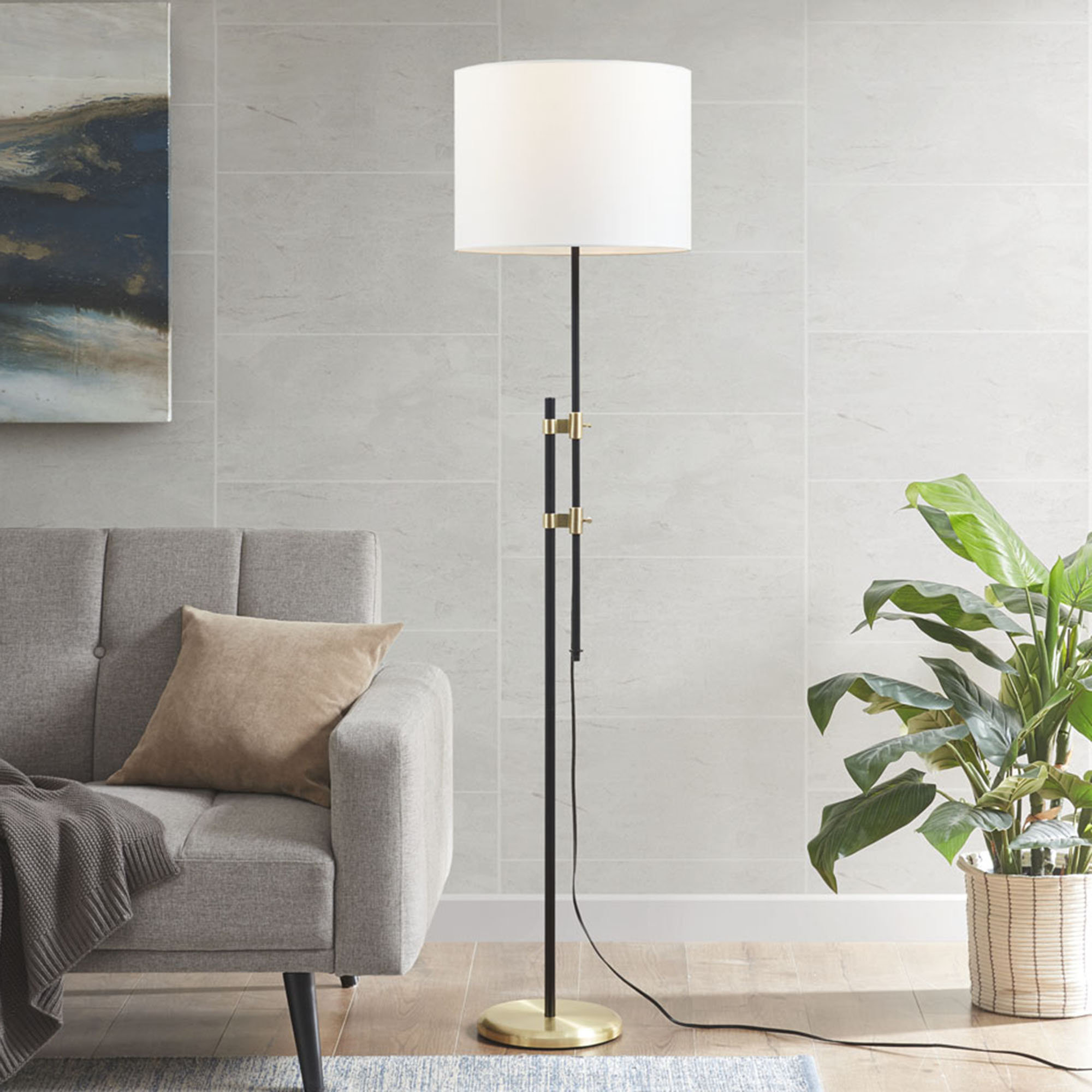The image captures a crisp and clear view of a tastefully designed living room, showcasing a muted and lovely photography style. The focal point is a tall floor lamp with a cream cylindrical lampshade, a black stem adorned with gold clasps, and a sturdy gold base. To the left of the lamp, half of a cozy, soft gray upholstered couch with clean lines is visible. The couch features a tan (almost orange) pillow and a dark gray (almost gray-brown) throw blanket draped over it. The couch partially rests on a thin gray area rug that covers the brown tile floor.

The back wall, which has a light gray tile or gray marble appearance, serves as a sophisticated backdrop. In the upper left-hand corner of the wall, there is an abstract painting with dark blue, white, and tan strokes. On the floor to the right of the lamp stands a potted plant in a wicker-like basket, positioned neatly on the brown tile floor. The overall arrangement creates a harmonious and inviting living space with a touch of modern elegance.